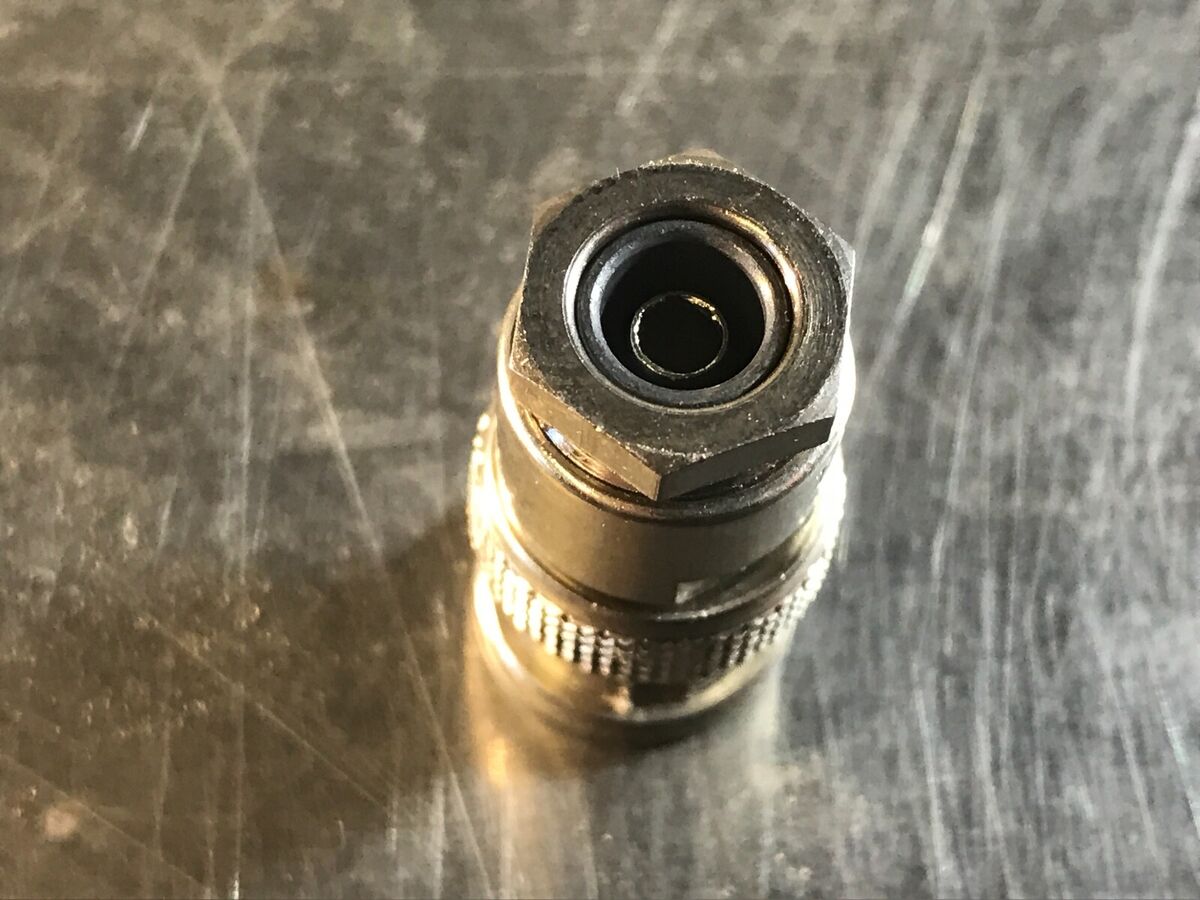The image is a full-color, square photograph featuring a metallic object, primarily a slightly gold bolt, with multiple sections that give the appearance of several bolts stacked together. The top of the bolt, which is hexagonal with six sides, is in sharp focus, while the lower part fades into a blur. The middle portion of the bolt is roundish with a couple of metallic circular tubes inside, while the bottom appears to have a grip texture, suggesting its functional aspect for turning. The backdrop showcases a very scratched-up metal surface, which might be a gray granite table. The surface is brighter on the right side and darker on the left, likely due to a light source reflecting off the top part of the bolt, highlighting its metallic sheen.